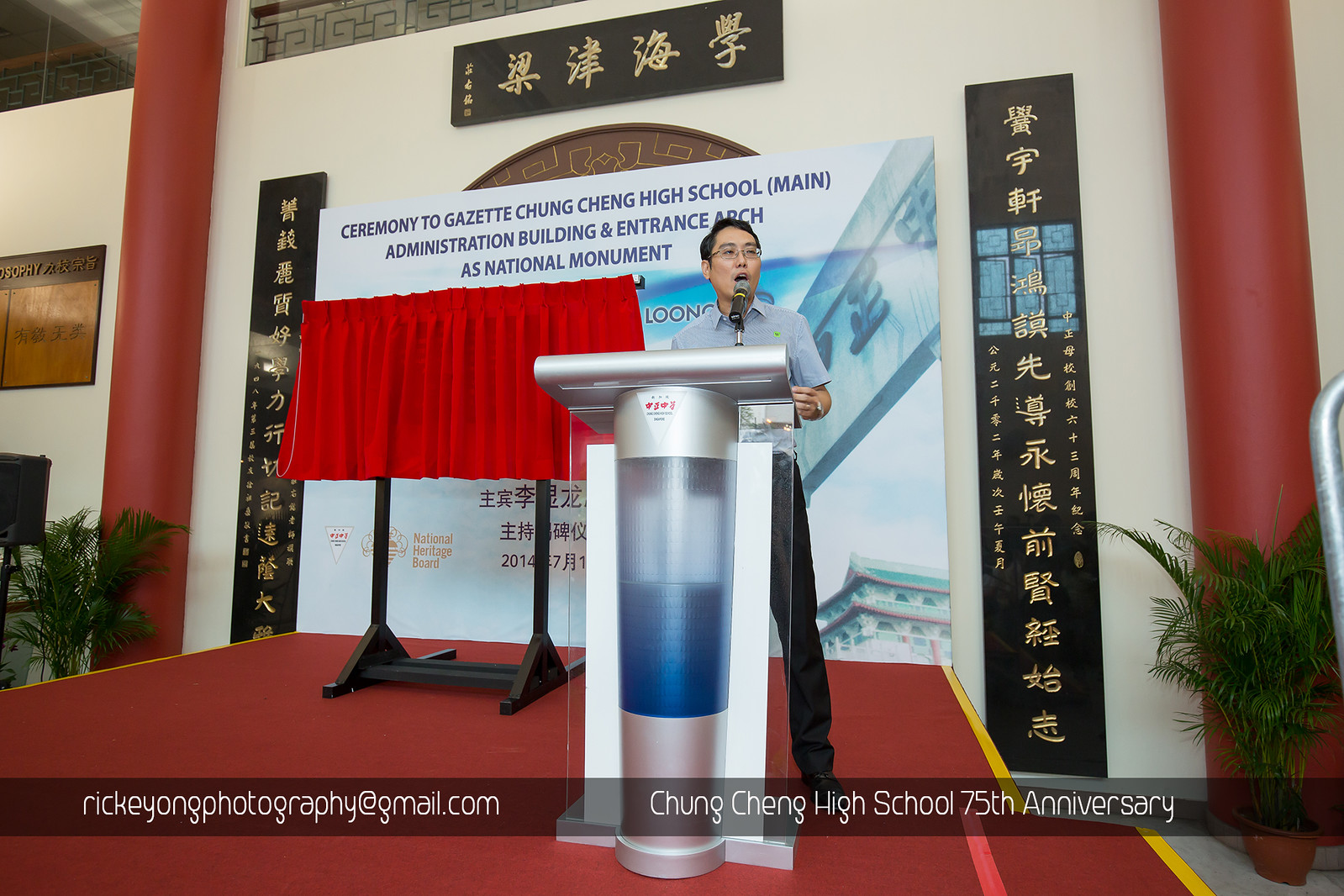A man with short black hair, glasses, and a short-sleeved gray button-up shirt is standing slightly to the right side of a futuristic, silver podium on a stage with dark red carpet. The podium features a hollow, cylinder-like structure with a semi-transparent middle section, showcasing a clear pipe inside. The man addresses the audience through a microphone, which has a silver end and a yellow circle near the tip, mounted on a silver piece in front of him. Behind the man, a white sign reads "Ceremony to Gazette Chung, Chung Cheng High School Main Administration Building and Entrance Arch as National Monument." This sign is partially obstructed by the man and flanked by thin, tall black columns with gold Asian characters. Above the sign, a black rectangle also displays gold characters. Below, a gray bar states "Ricky Young Photography at gmail.com" and "Chung Cheng High School 75th Anniversary." To either side of these black columns are red pillars extending to the ceiling, each accompanied by a short green plant. Additionally, there is a red curtain covering an object on a stand, suggesting an upcoming unveiling. Steps with yellow strips lead up to the stage on the right side.